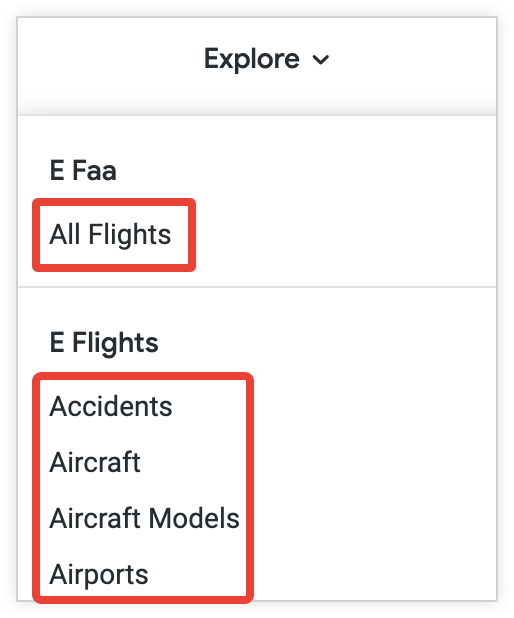The image features a small, white square pop-up window with a clean design. At the top center of this window, the word "Explore" is prominently displayed in black font. On the left side, there are two distinct categories, each accompanied by several subcategories. 

The top category, labeled "EFAA," has a single subcategory titled "All Flights," which is highlighted with a red outline. Below it, the second category, "E-Flights," contains four subcategories: "Accidents," "Aircraft," "Aircraft Models," and "Airports." These four subcategories are collectively enclosed within a red square outline. 

The entire window has a white background, providing a clear contrast to the black text, enhancing its readability. The structured layout and minimalist color scheme emphasize the organization and hierarchy of information within this interface element.